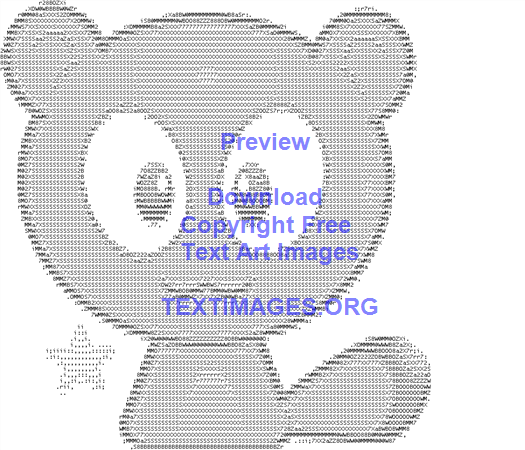The image is a detailed ASCII art graphic featuring a cartoon-like creature composed entirely of black computer text characters against a white backdrop. The creature has a big, circular head with distinct round ears on either side and prominent oval eyes with black irises placed close together. Below its smiling face, the body is triangular, resembling a beaker, and it has a teardrop-shaped tail extending to the right. Adjacent to the left side of the creature, there is a five-pointed star. Overlaying the image in blue text are the words: "preview, download, copyright-free, text art images, textimages.org."